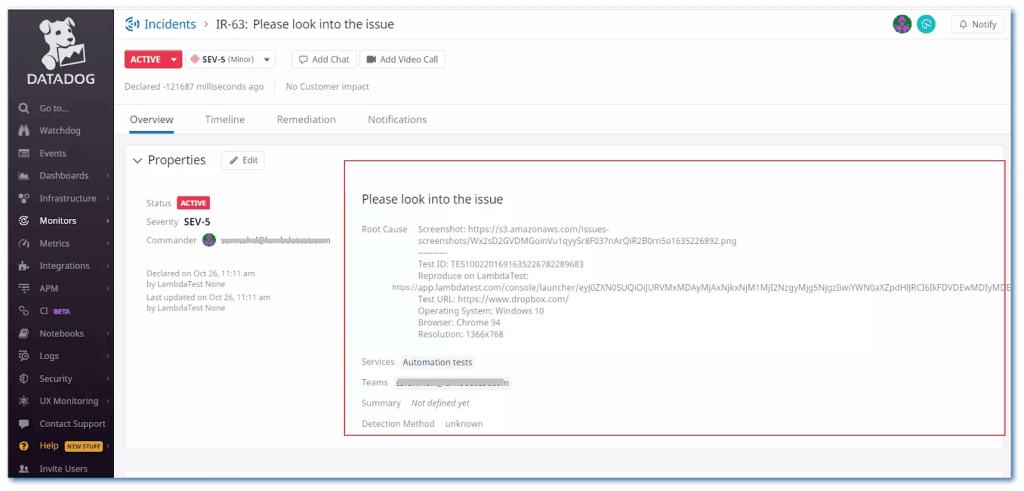This is a detailed screenshot of a program or website interface. 

On the left side, there is a dark grey vertical sidebar featuring a series of navigational icons and labels in white. At the top of the sidebar, a distinctive white icon depicts a dog holding a picture, labeled "Data Dog." Below this are multiple sidebar options arrayed vertically:

- A magnifying glass labeled "Go To."
- Binoculars labeled "Watch Dog."
- A calendar labeled "Events."
- A chart labeled "Dashboards."
- An icon with three white circles and one black circle labeled "Infrastructure."
- An arrow labeled "Monitors."
- A speedometer labeled "Metrics."
- A puzzle piece labeled "Integrations."
- Lines of text labeled "APM."
- An infinity symbol labeled "CI," marked "Beta" in purple text next to it.
- A book labeled "Notebooks."
- A magnifying glass over lines of text labeled "Logs."
- A shield labeled "Security."
- A virus icon labeled "UX Monitoring."
- A message box labeled "Contact Support."
- A question mark in gold or mustard yellow, labeled "Help," followed by a gold box labeled "New Stuff."

Beneath these options, there are two icons of people labeled "Invite Users."

Occupying the bulk of the page to the right of the sidebar is a content area with a white background. At the top, in blue text, it says "Incidents." Next to this, an arrow points to the right toward the text "IR-63, please look into the issue."

Underneath this heading, there are several interactive buttons:
- A red button with white text that says "Active."
- A white box labeled "SEV-5" with the word "Minor" in parentheses.
- A button labeled "Add Chat."
- A button labeled "Add Video Call."

This detailed layout enables efficient navigation and management of various functionalities within the program or website.